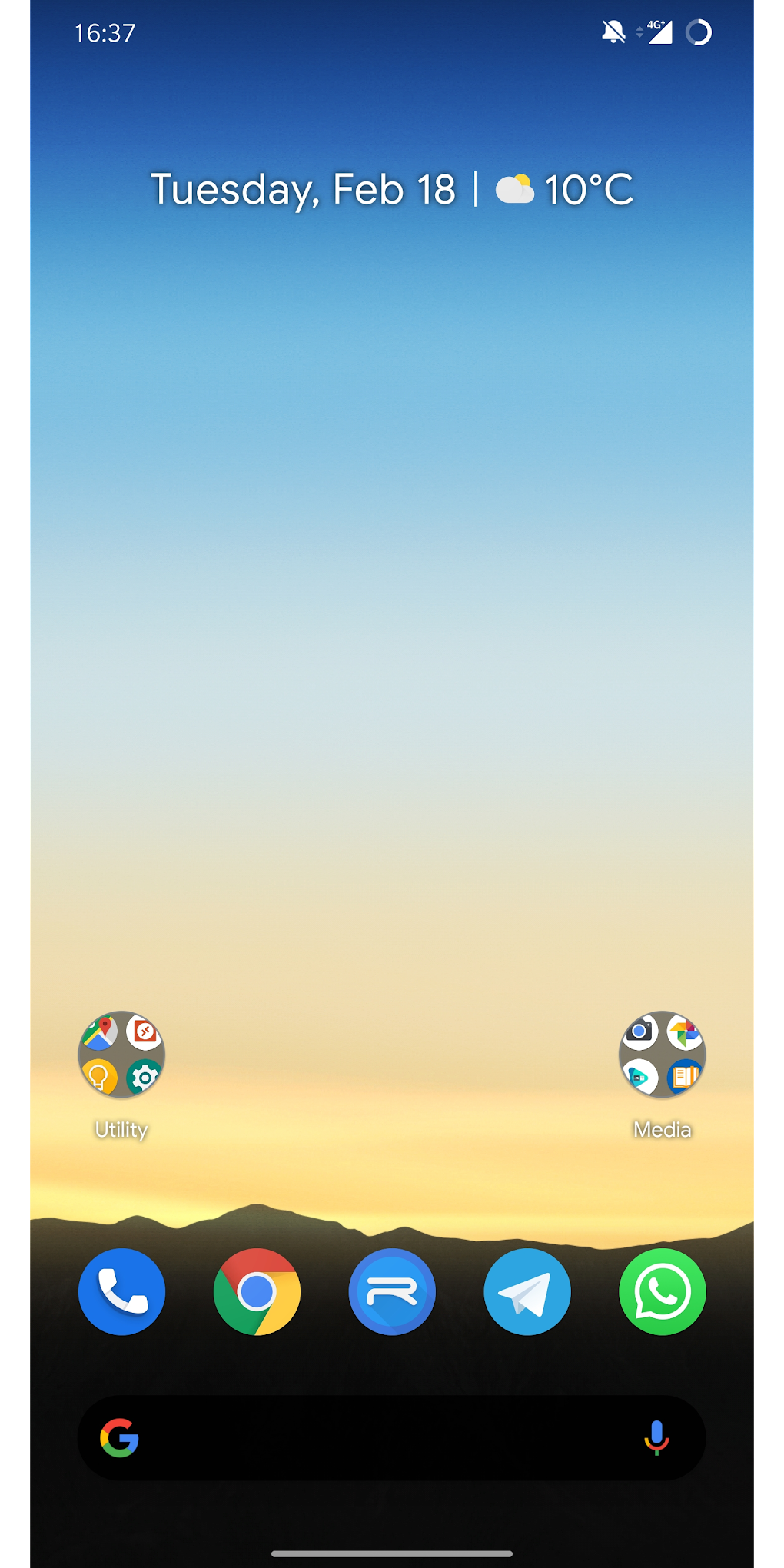This is a screenshot of a smartphone displaying various details. The time shown is 16:37. In the upper right corner, three icons are visible: a bell, a signal indicator showing "4G," and a loading circle. Below these, the date is displayed as Tuesday, February 18.

The weather widget shows a partly cloudy day with a sun icon and a temperature of 10 degrees Celsius. The background image features a gradient sky that transitions from dark blue at the top to light blue, then to white, pink, and finally orange, with a mountain silhouette at the bottom.

On the home screen, there are five icons positioned above the mountain silhouette: a telephone icon, the Google app, an app with an "R" in the middle, a circular icon with a paper airplane, and a green icon featuring a telephone and a speech bubble. Above these, two folder icons are visible: one labeled "Utility" containing four apps including Settings and Google Maps, and another labeled "Media" containing four apps including Google Photos.

At the bottom of the screen, there's a Google "G" logo next to an oval, black search bar with a microphone icon on the right.